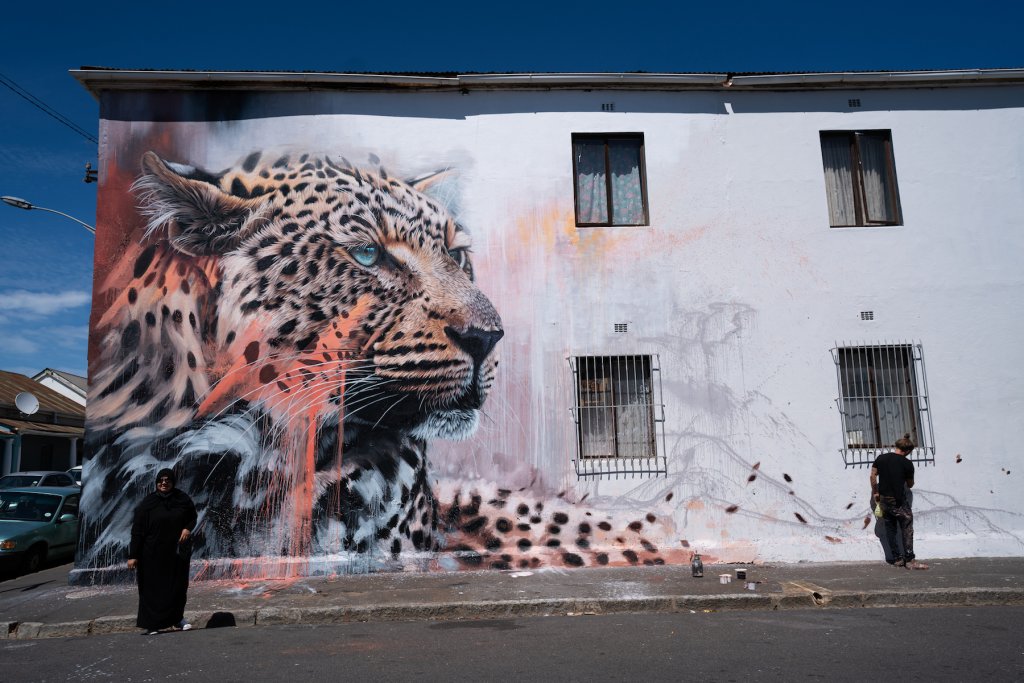In the photo, a two-story apartment building features prominently with a detailed and striking mural of a golden-yellow leopard adorned with black spots that spans a portion of its side wall. The mural, which captivates the viewer with its lifelike quality, is in progress, with an artist actively painting it on the right side near the first-floor window, where his equipment is scattered nearby. This window, along with another on the ground floor, is protected by wire gates, while two more windows are visible on the second floor. In front of the mural, there stands a woman dressed entirely in black, including a black head wrap or hijab. The street in front of the building appears dirty, with noticeable paint spills on the ground. The sky is clear with a few clouds, indicating that the photo was taken in the middle of a sunny day.